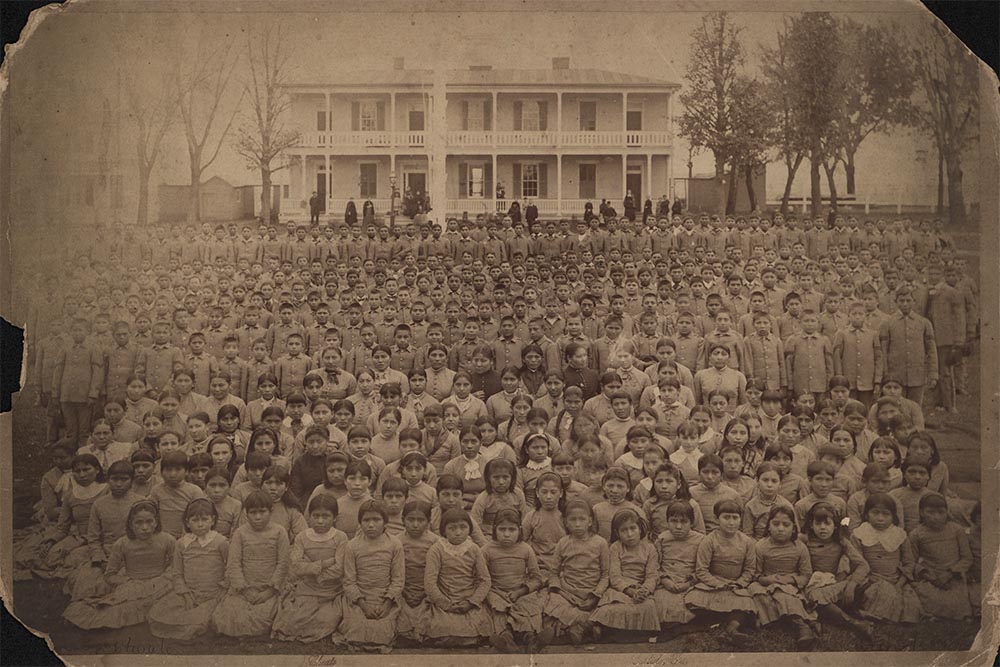This vintage, black-and-white photograph captures a large group of school children in front of a white, two-story building, likely a school. The children, who appear to be a mix of Hispanic and native heritage, are arranged with girls sitting in the front wearing gowns, and boys standing behind them in proper school shirts and trousers. In the back rows are older boys, likely from senior classes, and adults dressed in black. The background reveals a building with two floors, flanked by trees on the left and right sides, further emphasizing the historical context of the early 1900s. The absence of text in the photo leaves the scene open to interpretation but highlights a moment of educational gathering possibly aimed at cultural assimilation.